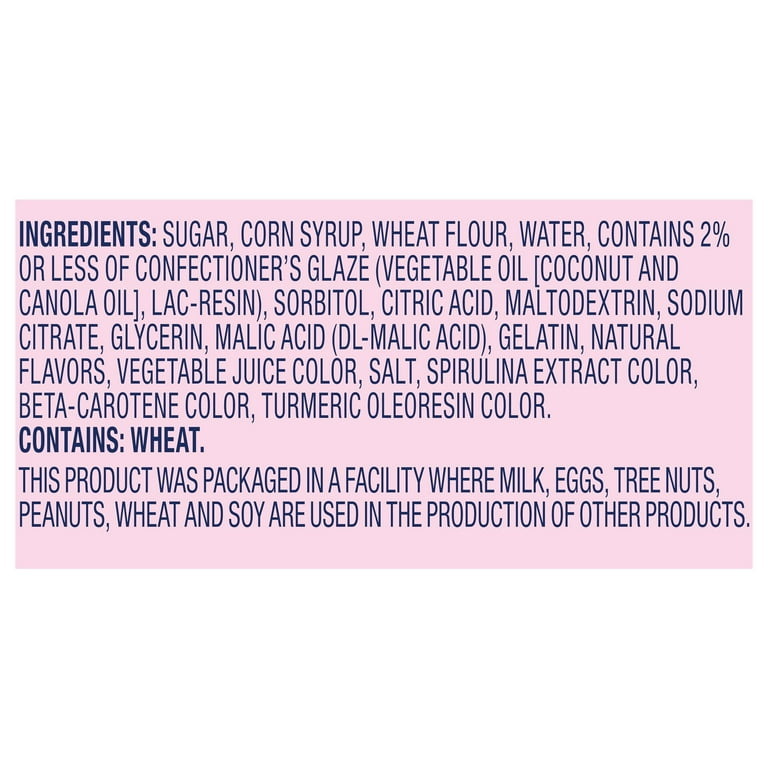This image depicts a horizontally aligned rectangular nutrition label set against a light pink background with no border. The detailed ingredients list is written in all caps using dark blue letters. At the upper left corner, the bolded word "INGREDIENTS" introduces the list. The ingredients include: sugar, corn syrup, wheat flour, water, and then a note stating "contains 2% or less of" followed by confectioner's glaze, vegetable oil (specifically coconut and canola oils), lac resin, sorbitol, citric acid, maltodextrin, sodium citrate, glycerin, malic acid, DL malic acid, gelatin, natural flavors, vegetable juice color, salt, spirulina extract color, beta-carotene color, and turmeric oleoresin color. Below this comprehensive list, the word "CONTAINS: WHEAT" is also bolded. Lastly, the label includes a warning in regular font, stating, "This product was packaged in a facility where milk, eggs, tree nuts, peanuts, wheat, and soy are used in the production of other products." Outside the image, the background is solid white.